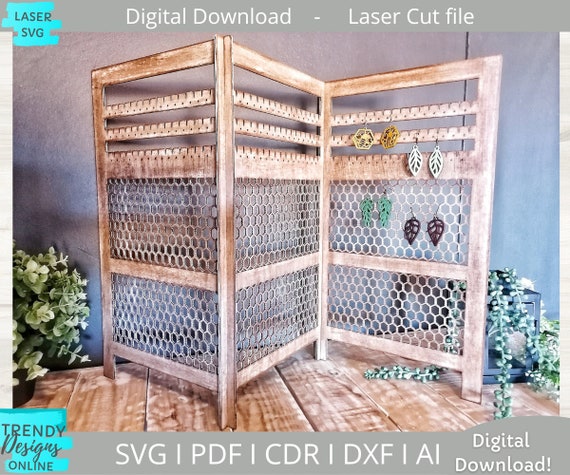This image depicts a folded, honeycomb-structured wooden earring holder positioned indoors. The main focal point is the earring holder, which consists of three interconnected, foldable panels adorned with slats and mesh caging for hanging earrings. Each panel features a brown trim and multiple slots and holes for earring placement. On the rightmost panel, four pairs of earrings are showcased: a yellow hexagon-shaped pair, white leaf-shaped ones, green feather-like earrings, and another pair of brown leaf-shaped earrings.

The earring holder is set against a gray wall with a wooden floor beneath it, suggesting an indoor environment. To the right and behind the holder, there's a square pot with three vines extending from it. Another plant is partially visible at floor level on the right side. The image has a somewhat blurry, computer-generated appearance, with the main colors being the brown wood of the holder, the wooden floor, and the gray wall.

Text elements are also present in the image. At the top left, within a blue, puzzle-piece-like icon, it reads "laser SVG," while a gray banner across the top states "digital download laser cut file." In the bottom left, another puzzle-piece icon displays "trendy designs online," and below it, the gray banner lists various file formats including "SVG, PDF, CDRI, DXF, AI," with a notation of "digital download" in white lettering.